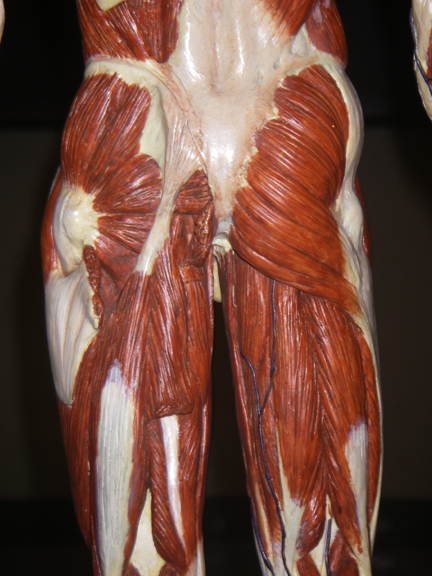The image depicts a model of a human man's lower torso and legs, showcasing the intricate musculature from the waist down to just above the knees. This anatomical model, similar to those found in medical offices, reveals the posterior view of the buttocks and the back of the thighs in vivid detail. The exposed muscles are depicted in a dark, bloody red color, appearing sinewy and mechanical, with interspersed tendons and other anatomical structures highlighted in white. A few blue veins are visible, particularly running down the inside of the man's right leg. The stark contrast against a jet black background accentuates the anatomical details, making the red and white elements stand out more prominently.